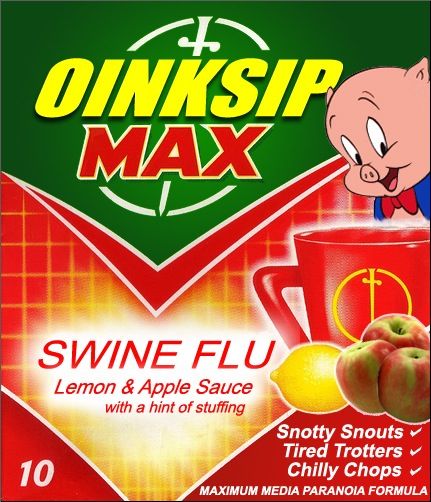The image depicts a satirical packaging design, primarily green and red, with vivid yellow accents and lettering. Dominating the top is an inverted green triangle with the text "OINKSIP" in bold, yellow letters, and "MAX" in red letters underneath. To the right of these words is an illustration of Porky Pig, smiling, with a red mug below him. The mug features a gold circle on its front. Next to this, a segment in red print on a white background reads: "SWINE FLEW LEMON AND APPLE SAUCE with a hint of stuffing." Adjacent to this, there are images of a lemon and three apples. In the lower left corner, the number "10" is printed in white on a red background. On the lower right, also in white on red, are the phrases "SNOTTY SNOUTS," "TIRED TROTTERS," and "CHILI CHOPS," each with a checkmark beside them. Below these phrases is the tagline "MAXIMUM MEDIA PARANOIA FORMULA."